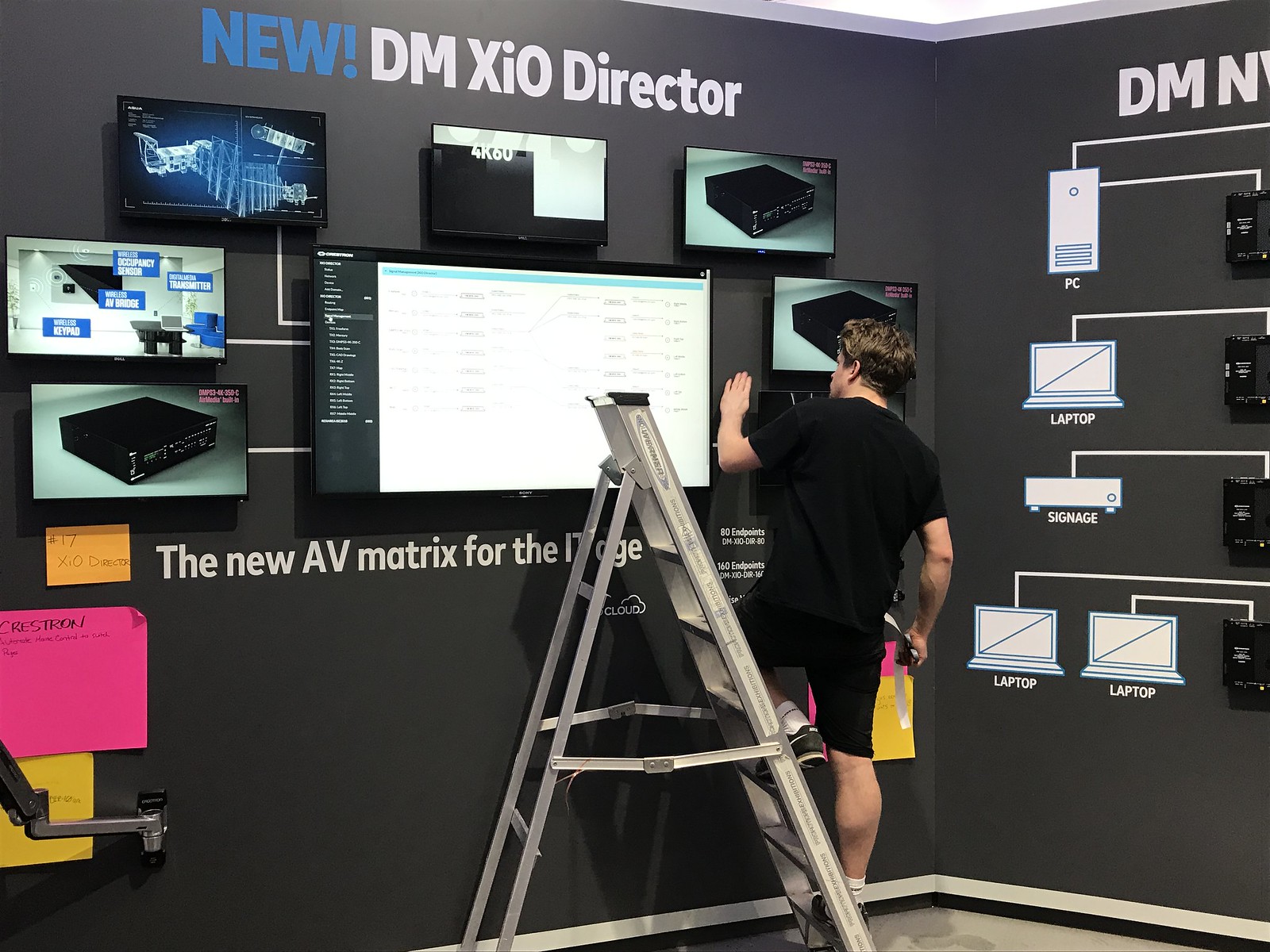In this image, a man dressed in a black t-shirt and black shorts is seen standing with one foot on a silver ladder, apparently affixing or adjusting objects on a large gray wall. The wall features various displays and advertisements, primarily focused on technology and electronics. Prominently displayed at the upper left is text reading "New DMXIO Director," along with a large TV screen that shows a white display and multiple connected components. Surrounding the TV are smaller monitors and pictures of different electronic devices such as a cell phone screen, multiple laptops, a PC, and a modem, suggesting a focus on connectivity and cloud technology. The caption "The New AV Matrix for the i7" can be partially seen near the TV. The bottom part of the wall has a white border above a white floor, leading to a corner of the room, which gives the impression that this may be an electronics store or a tech display setup. The man appears to be engaged in setting up or touching up the display on the wall.